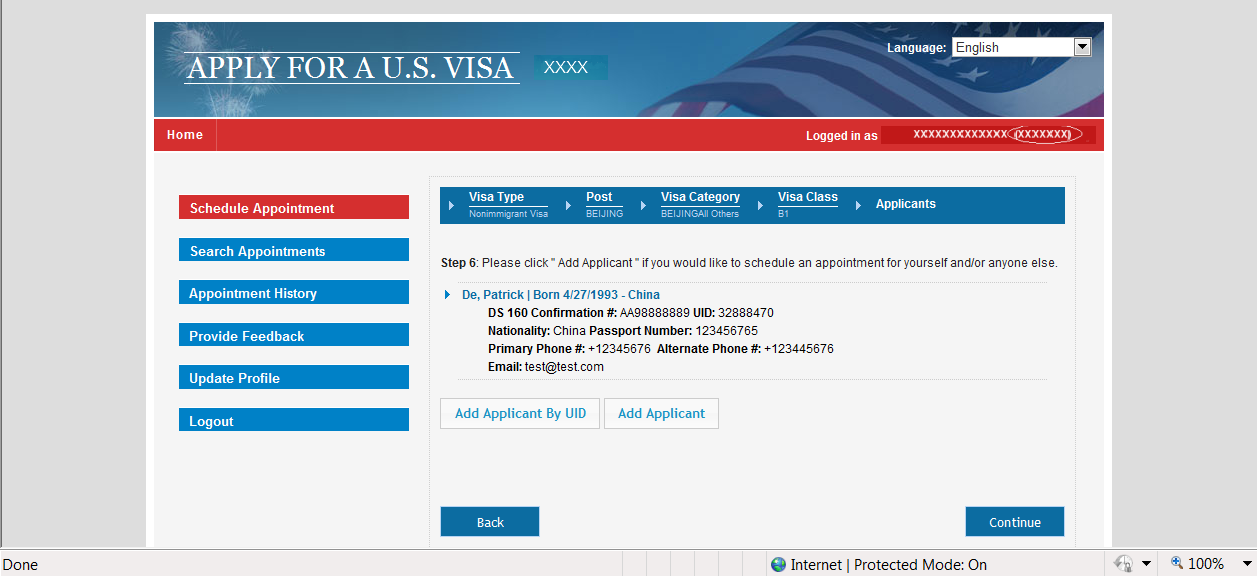The image depicts a web page for applying for a United States visa, prominently featuring a red, white, and blue color scheme symbolic of the American flag. The top navigation bar is blue with an integrated portion of the U.S. flag, setting the patriotic theme. Directly beneath this is a red stripe where users can log in, labelled 'Home.'

The overall page background is white, complemented by additional blue and red bars, contributing to the cohesive red, white, and blue design. The interface offers several functionalities: scheduling an appointment, searching for appointments, viewing appointment history, providing feedback, updating profiles, logging out, adding an applicant by UID, and selecting visa types, categories, and classes. 

The displayed content shows that the user is currently on 'Step 6: Add an Applicant,' an essential step for those looking to schedule a visa appointment for themselves or others. Although the page lists a name and a phone number, these details are confirmed to be fake, ensuring no violation of personal information.

The entire interface is presented within a gray background, encapsulating the functional elements inside a distinct rectangular frame, maintaining a clear and organized layout.